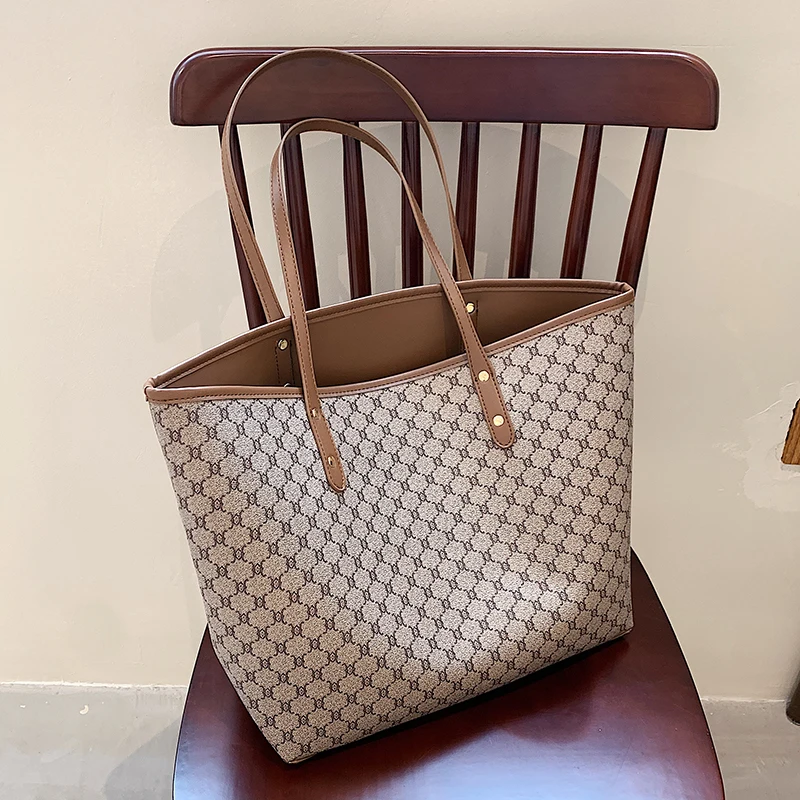This close-up photograph captures a vintage mahogany wooden chair, placed in a room with a light pink vanilla-colored wall and gray wooden flooring. The chair, which is simple in design without armrests, features a backrest comprised of eight vertical cylindrical poles, topped with a curved rectangular bar. Bathed in light, the base of the chair appears slightly white due to the illumination. Resting on the chair is a light brown ladies' handbag adorned with a diamond-shaped, beehive-like graphic pattern. The handbag has a light brown body with a brown leather upper border and two brown straps, each fixed with golden yellow buttons. The detailed textures and colors of both the chair and the handbag are accentuated by the soft background and lighting, creating a harmonious and detailed vignette.